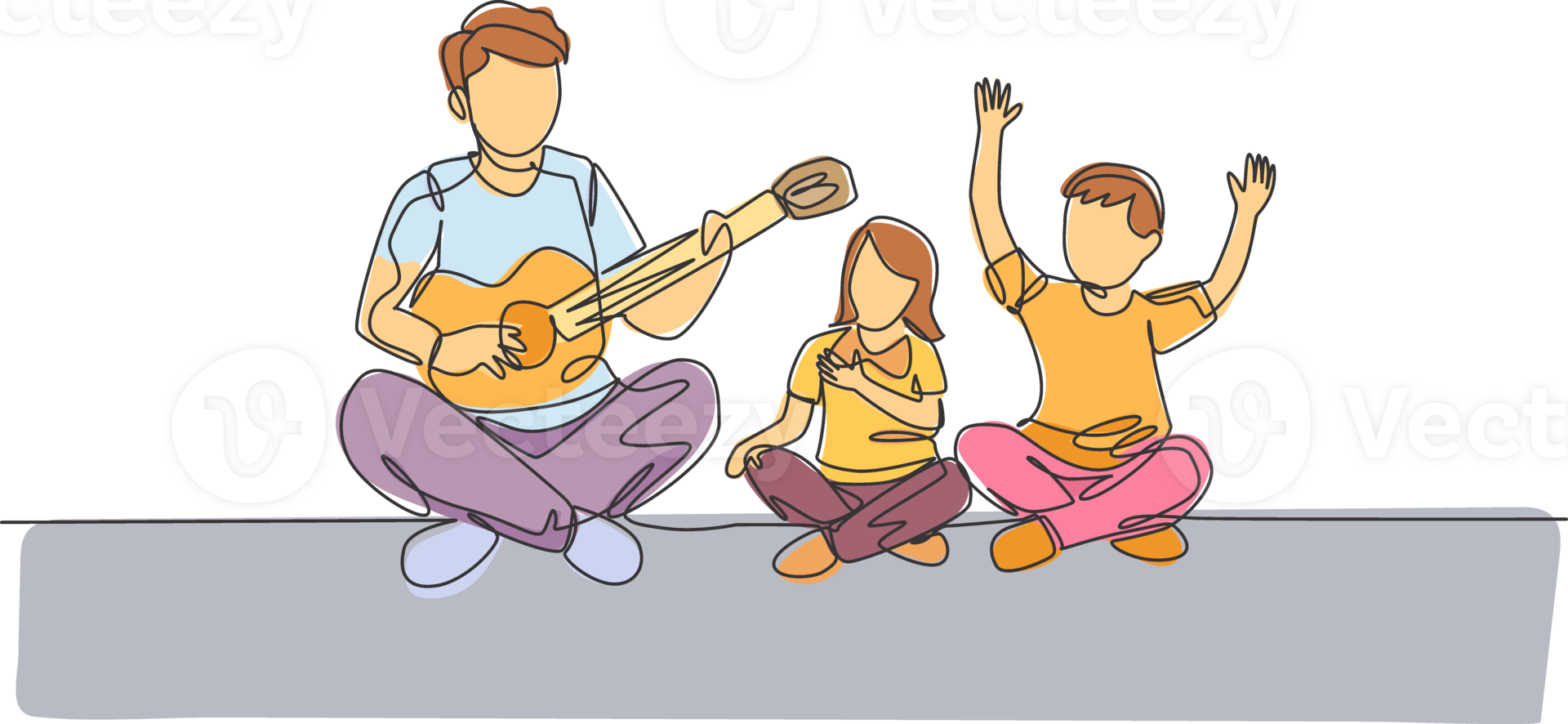This image is a stylized, cartoon-like illustration depicting a family scene. On the left side, there's a man, presumably the father, playing an acoustic guitar. The characters are rendered in simple line art and colored with vibrant shades. The father, sporting brown hair, wears a light blue shirt, purple pants, and blue shoes. To his right, a young girl with brown hair is wearing a yellow shirt, dark purple pants, and orange shoes, while a young boy, also with brown hair, is dressed in an orange shirt, pink pants, and orange shoes. The children are seated cross-legged, looking and listening intently to their father. Notably, the characters lack facial features, adding to the stylized and abstract nature of the illustration. They are seated on a gray surface, with a stark white background, emphasizing the simplicity and focus on the characters themselves.